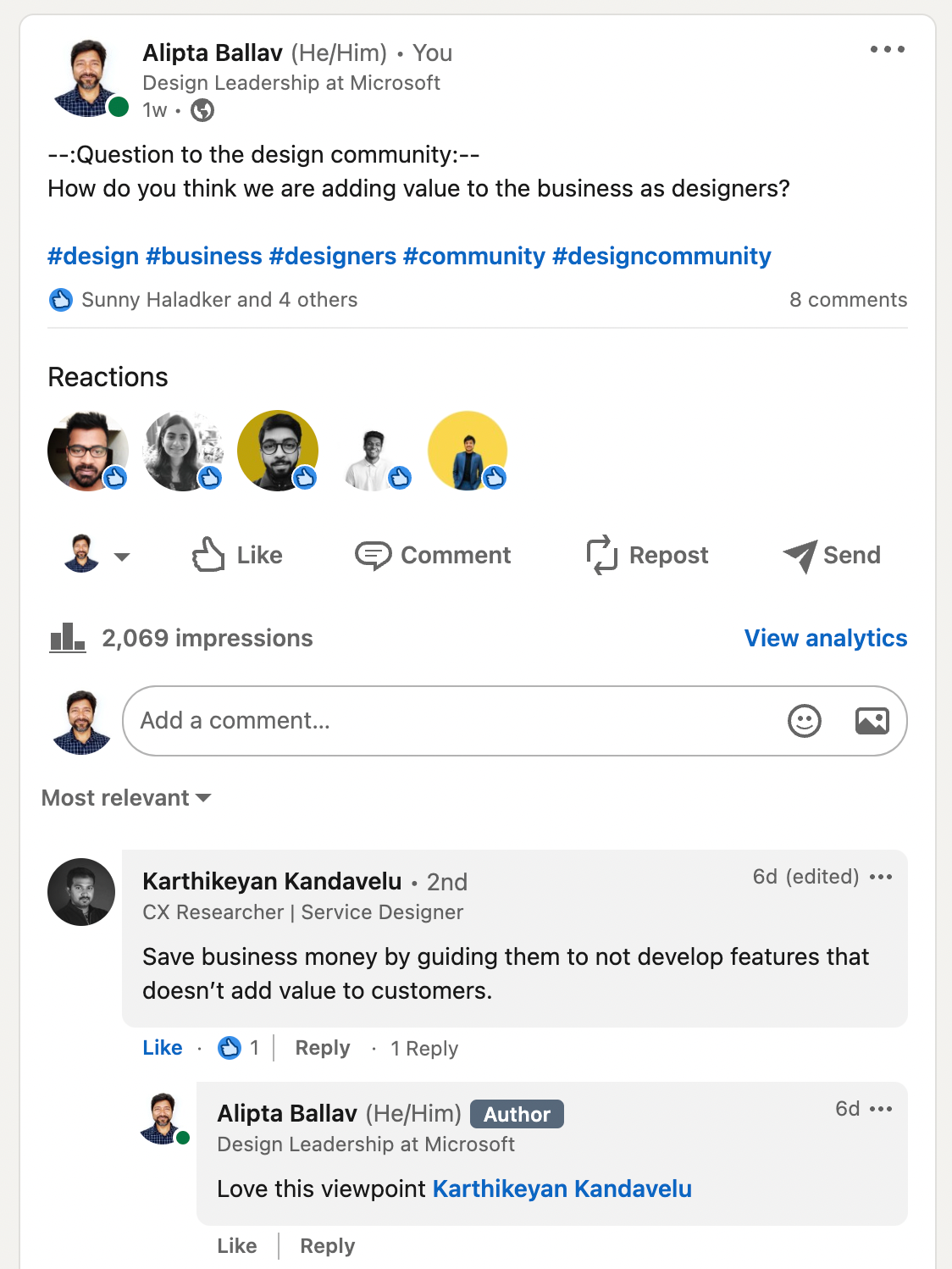This is a social media post screenshot featuring a design-related inquiry. The post is visually framed by a light grey background with a central white panel that has slightly rounded corners, giving it a modern and clean appearance.

### Upper Section:
- **Profile Picture**: A man with a beard and short hair is displayed at the top left, accompanied by a green dot indicating online status.
- **User Information**: To the right of the profile picture, the user information is organized as follows:
  - **Name**: Bolded text "Alipta Balav" with a grey parenthetical notation "(he/him)" to the immediate right.
  - **Additional Info**: A grey dot follows the pronoun notation, then the text "you," indicating the viewer's connection to the poster.
  - **Professional Title**: Below the name, it reads "Design Leadership at Microsoft" in smaller text.
  - **Post Timing**: The text "1W" (indicating the post was made one week ago), followed by a grey dot and a medium grey globe icon.

### Post Content:
- **Question**: Black text with dashes and colons demarcates the main question to the design community: "How do you think we are adding value to the business as designers?"

### Hashtags:
- Multiple hashtags in blue text are listed below the question:
  - #design
  - #business
  - #designers
  - #community
  - #designcommunity

### Interaction Summary:
- **Initial Interactions**: In light grey text, it says "honey halad ker and 4 others,” indicating individuals who have interacted with the post.
- **Like Button**: A blue circle with a white thumbs-up icon is positioned to the left of the interaction summary.
- **Comments**: Light grey text denotes "8 comments" to the right.

### Additional Information:
- A thin light grey line separates the main post content from further information below.
- **Reactions**: Label "Reactions" in the top left, showing five profile pictures, each marked with a blue circle and a white thumbs-up icon at its bottom right.
- **Post Options**: Below the reactions, options such as "Like," "Comment," "Repost," and "Send" are accessible.
- **Post Analytics**:
  - On the left: "2069 impressions."
  - On the right: "View analytics" in blue text.
- **Comment Section**: Located beneath the post analytics for further reading and engagement.